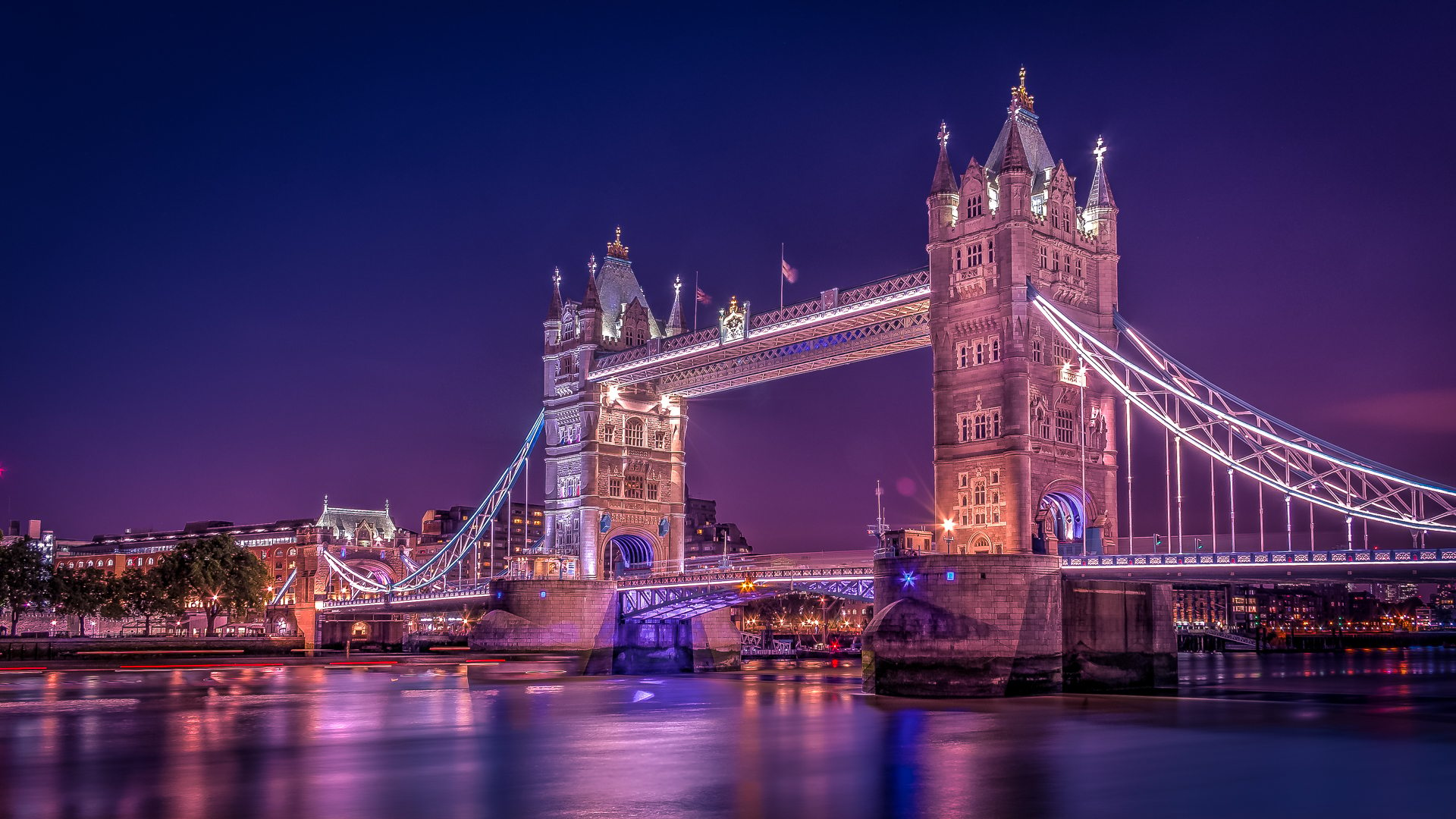The image depicts a stunning and stylized nighttime view of London's iconic Tower Bridge. Dominating the center of the frame, the bridge is beautifully lit, with a symphony of bright white, purple, and pink lights that create a vibrant and enchanting atmosphere. The illumination artfully cascades from the bottom to the top of the structure, highlighting the impressive architecture and casting intriguing reflections on the river below. The image may be a time lapse, as the water appears blurred, capturing the continuous flow and reflections of the city lights in shades of purple, yellow, and blue.

The sky transitions from a purple hue at the horizon, suggesting the remnants of sunset, to a darker navy blue as it ascends, devoid of stars or planets. Flanking the bridge, we see the silhouettes of various buildings and pockets of green trees along the riverbank, all accentuated by the city's ambient glow. The two towers of the bridge are connected by both an upper walkway with a crown image flanked by Great Britain flags, and a lower level bridge designed for street traffic, with intricate metal trusses and further purple light illumination.

Overall, the scene is a meticulously detailed and photorealistic capture of Tower Bridge at night, encapsulating the serene yet lively essence of London, beautifully reflected in the tranquil river.